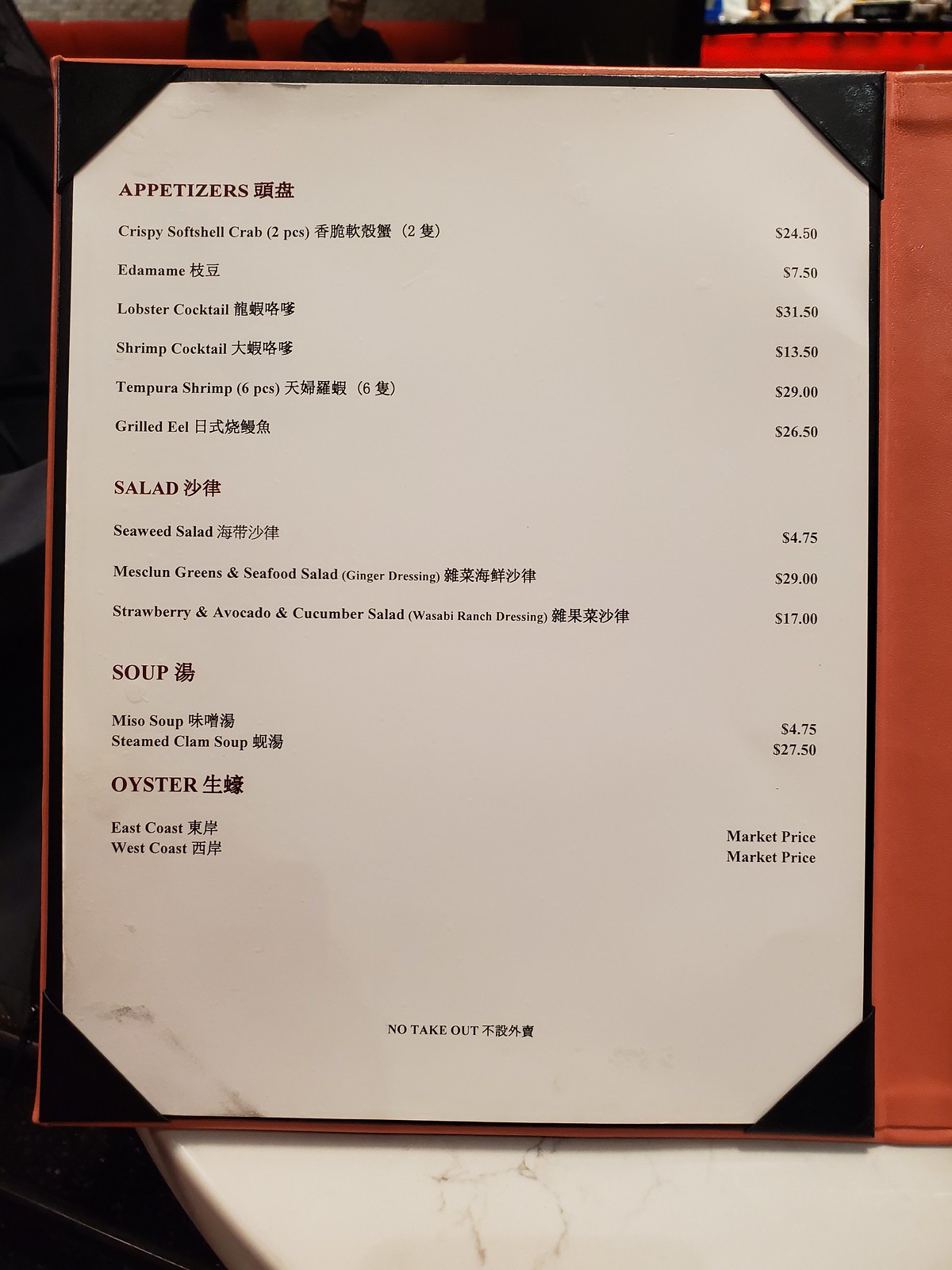The image features a vertically oriented, color photograph of the last page of a high-quality, trifold menu. The menu rests on a round marble table, and the background and back page are crafted from an orange, leather-like material. Each corner of the menu has leather insets designed to hold the page securely, allowing for easy updates to the menu items.

The menu itself is bilingual, featuring English and an unspecified Asian language. It is organized into four distinct sections: Appetizers, Salads, Soups, and Oysters. In the appetizer section, items such as Lobster Cocktail, Shrimp Cocktail, and Grilled Eel are listed. The salad section includes options like Seaweed Salad and a Strawberry, Avocado, and Cucumber Salad. The soup section offers choices between Miso Soup and Steamed Clam Soup. The oyster section distinguishes between East Coast and West Coast oysters, priced at market value. Other prices on the menu range from $7.50 to $29.00, reaching up to $27.50 for specific items. At the bottom center of the page, a note specifies that take-out service is not available.